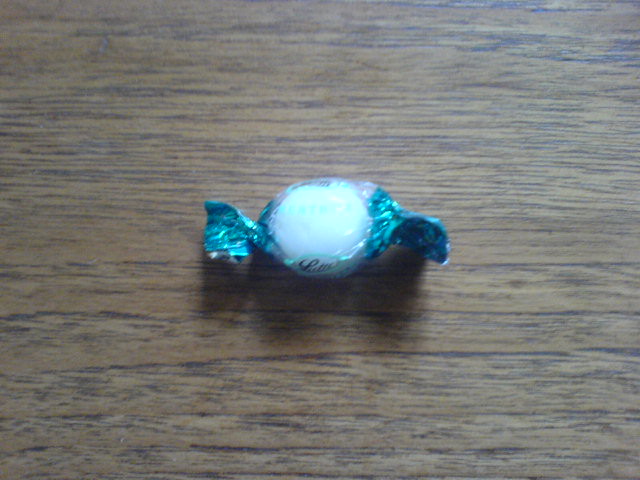A detailed photograph captures a solitary, round piece of hard candy resting on a plain brown wooden tabletop, which features distinct black grain patterns running horizontally. The candy is encased in a blue wrapper that is twisted closed at both ends, although the right end appears half unwrapped, suggesting a partial attempt to open it. The wrapper bears black script-like writing that somewhat resembles the Lindt logo, though Lindt is known primarily for chocolates. The focus of the image is tight on the candy, with no other objects or identifying features visible in the frame, emphasizing the lonely and striking simplicity of the scene.